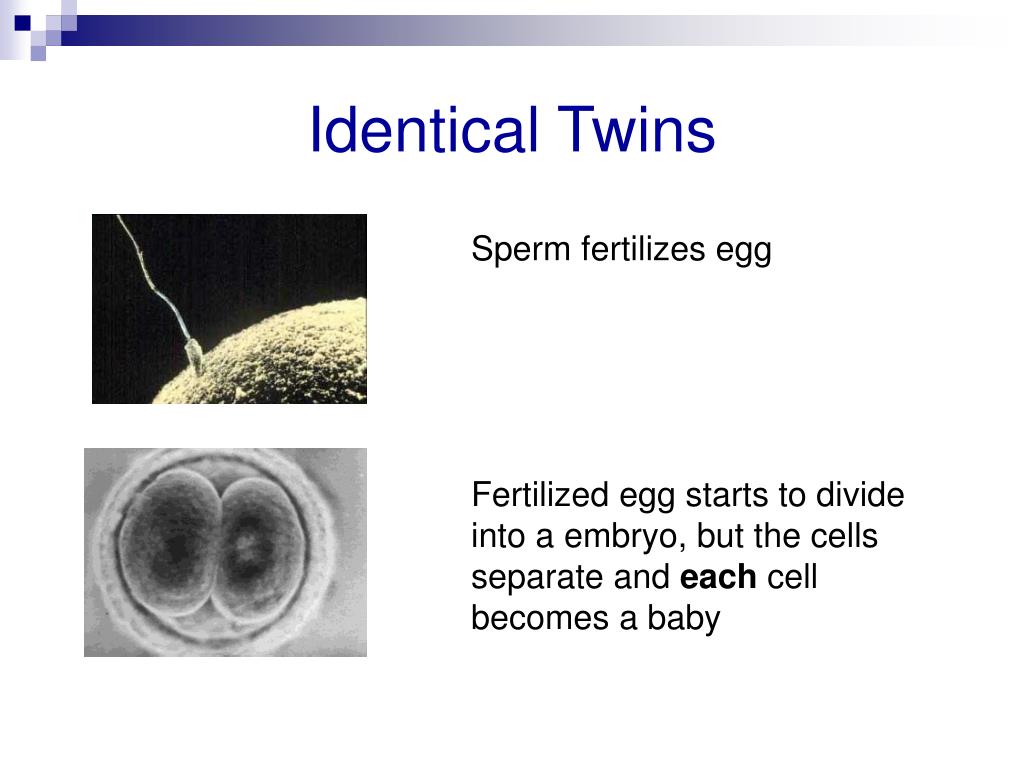The image is an educational slide, predominantly set against a white background. At the top, there is a horizontal blue gradient bar that fades from dark blue on the left to light blue and then to white on the right. This bar includes a small, pixelated section featuring a dark blue square among lighter blue and white squares. Below this gradient bar, centrally aligned, the title "Identical Twins" is written in a bold, dark blue font.

On the left side of the slide, there are two vertically stacked rectangular images. The upper image displays a diagram with a black background, showing a rounded body part connected by a string-like structure, followed by explanatory text on its right that reads, "Sperm fertilizes egg." Below this is a second image, black and white resembling an x-ray, with a round shape containing two darker oval figures within a gray background. To the right of this image, it states, "Fertilized egg starts to divide into an embryo, but the cells separate and each cell becomes a baby,” with "each" emphasized in bold. The background is white, and the text throughout the image is rendered in basic black.